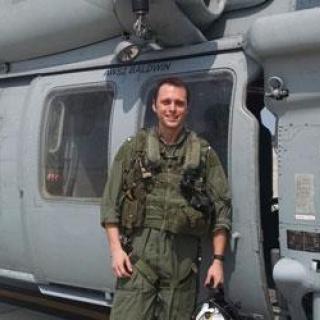In this detailed photograph, a tall, white man with dark brown hair, dressed in olive green, camouflage military fatigues, stands outside the side hatch of a gray aircraft, which appears to be a helicopter. The aircraft behind him, bathed in sunlight, features a large sliding door with two glass windows and the name "Baldwin" inscribed on it. The man, looking directly and smiling at the camera, is equipped with numerous pieces of gear attached to his vest and a large pack on his back, evidenced by visible straps. His sleeves are slightly rolled up, revealing a watch on his left wrist, and he holds what appears to be a helmet in his hand. He is positioned right in the middle of the frame, standing in front of the two doors of the aircraft.